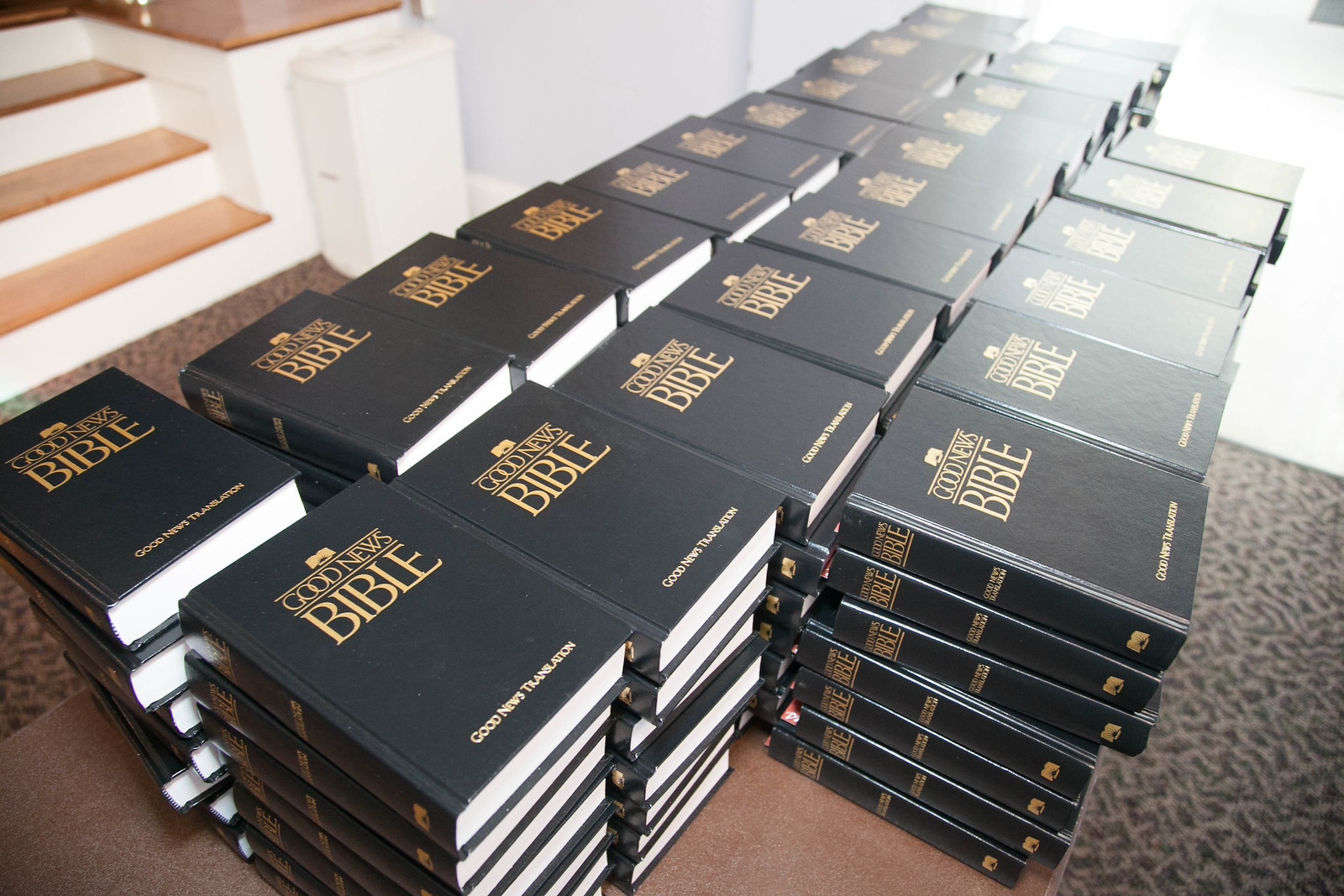The image depicts a color photograph of three rows of stacked Bibles, positioned at the bottom of a staircase. The Bibles, which appear to be identical, are black with gold writing on the front cover that reads "Good News Bible". At the bottom of each Bible, it further states "Good News Translation" in white text. These stacks are arranged in columns, each column consisting of seven or eight Bibles stacked vertically, and there are twelve or thirteen columns in total.

In the background, a white wall is visible alongside a staircase that ascends to the upper left side of the image. Each step of the staircase features a white front and a beige or brown wooden top. The floor around the Bibles includes a patterned carpet in tones of orangey-brown and black patterns on a light brown background, as well as sections of plain orangey-brown flooring. Additionally, a brown wooden table is partially visible, seemingly situated to the far right of the image.